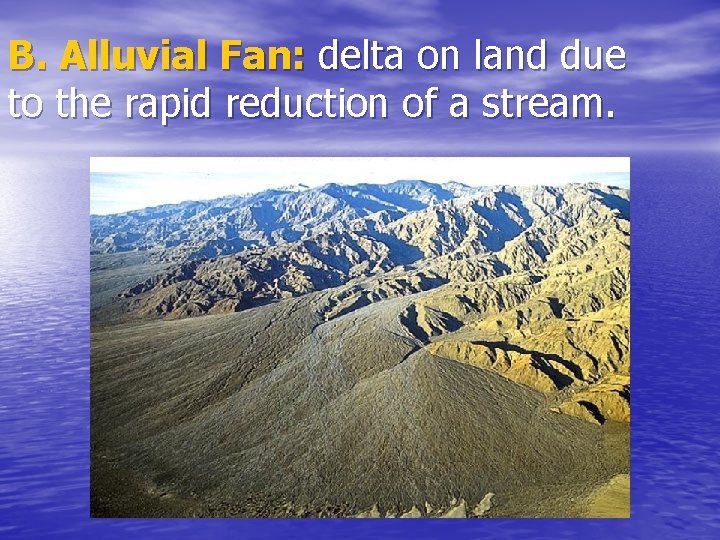The poster features a wide blue border with the heading "B. Alluvial Fan" in gold letters at the top. Beneath it, in white lettering, the text reads: "Delta on land due to the rapid reduction of a stream." The border is designed to look like rippling water, adorned with white clouds at the top. Centrally, the poster showcases a mountain range that appears drab with varying shades of brown and possibly green. The mountains in the foreground are a deeper and darker brown with smoother surfaces, whereas those in the background are lighter, rougher in texture, and exhibit yellow and dull gray tinges. The landscape includes hills, canyons, and scattered rocks but no visible trees.